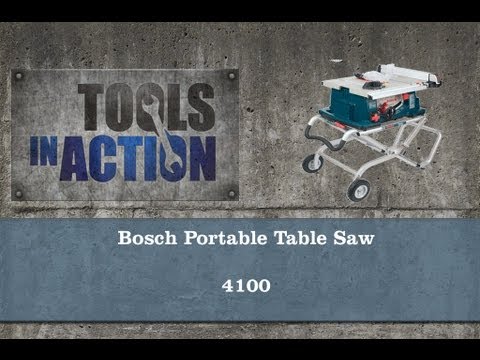The advertisement showcases a Bosch portable table saw, specifically the 4100 model, prominently displayed against a predominantly dark gray background. The ad features a small black frame with a darker gray fill, containing a prominent rectangle in the top left corner labeled "Tools in Action." The word "Tools" is in black, while "in Action" is in blue, with a wrench overlay covering part of the text. Adjacent to this label, on the right, is an image of the Bosch table saw, which is green with orange handles and knobs. The saw is mounted on a white cart with wheels, designed for easy maneuverability. Below the image, there's a blue background strip with the text "Bosch Portable Table Saw" and "4100" in white lettering, providing clear identification of the product.